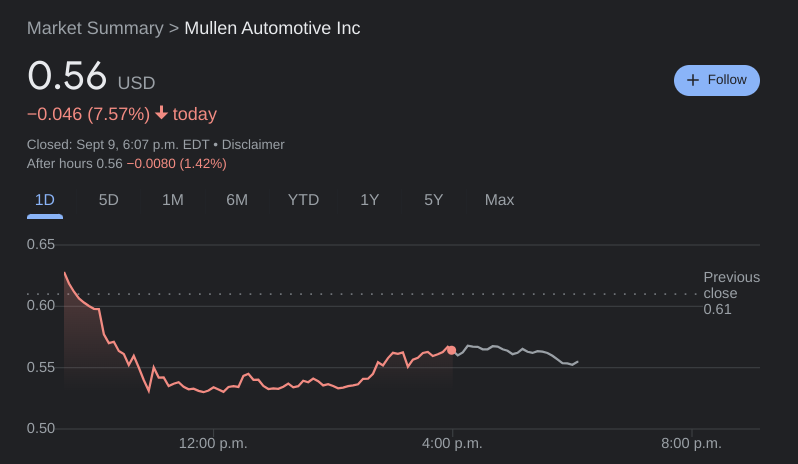This image is a screenshot of stock market information for Mullen Automotive, Inc., consistent with Google's stock display in night mode. The interface features a black background with white, light gray, and pink text. At the top, "Market Summary Mullen Automotive, Inc." is prominently displayed. Below this, the current stock price is shown as $0.56 USD, indicating a decrease of 7.57% for the day. Additional details about closed and after-hours trading are provided underneath.

The center of the image is dominated by a graph focusing on the stock's one-day performance. To the right of the graph are options for viewing different time frames: five days, one month, six months, year-to-date, one year, five years, and maximum.

The graph itself features a pink line representing the stock's price movement over the day. Starting near the top at $0.65, the line trends sharply downward to around $0.50 before fluctuating upwards inconsistently. The x-axis shows timestamps at 12 PM, 4 PM, and 8 PM. To the right side of the graph, text indicates the previous closing price, which was $0.61.